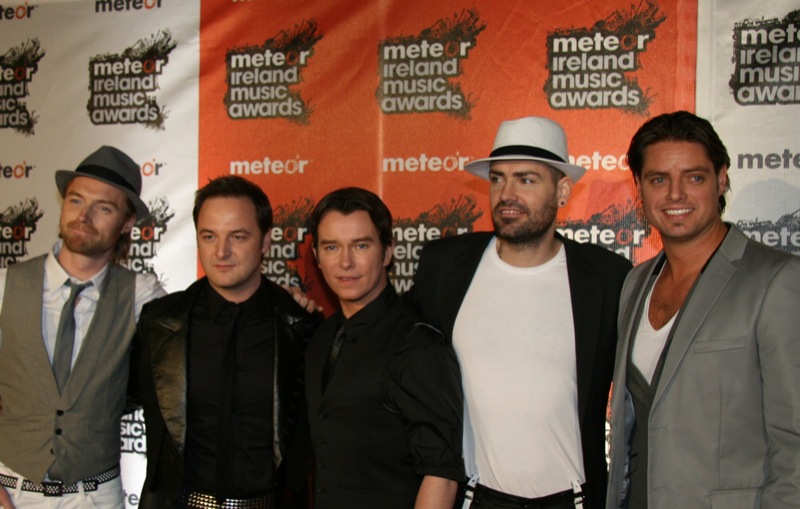In the image, five men are standing together with their arms around each other, appearing at the Meteor Ireland Music Awards. The backdrop features a white and orange sign with the awards’ name prominently displayed in white lettering. The first man on the left wears a brown vest, a white shirt, a brown tie, and a hat. The next individual is clad in a black suit. The third man sports a black shirt. Following him, the fourth man wears a white shirt with a black blazer and a white hat with a black band. The final individual is dressed in a gray blazer over a white shirt. The group is posed, looking in various directions, with most glancing towards an off-screen camera. The image captures their diverse attire, featuring elements like ties, jackets, and hats, suggesting they might be part of a music group. The setting of the photograph is indeterminate, giving no clear indication if it was taken indoors or outdoors, or whether it’s day or night.